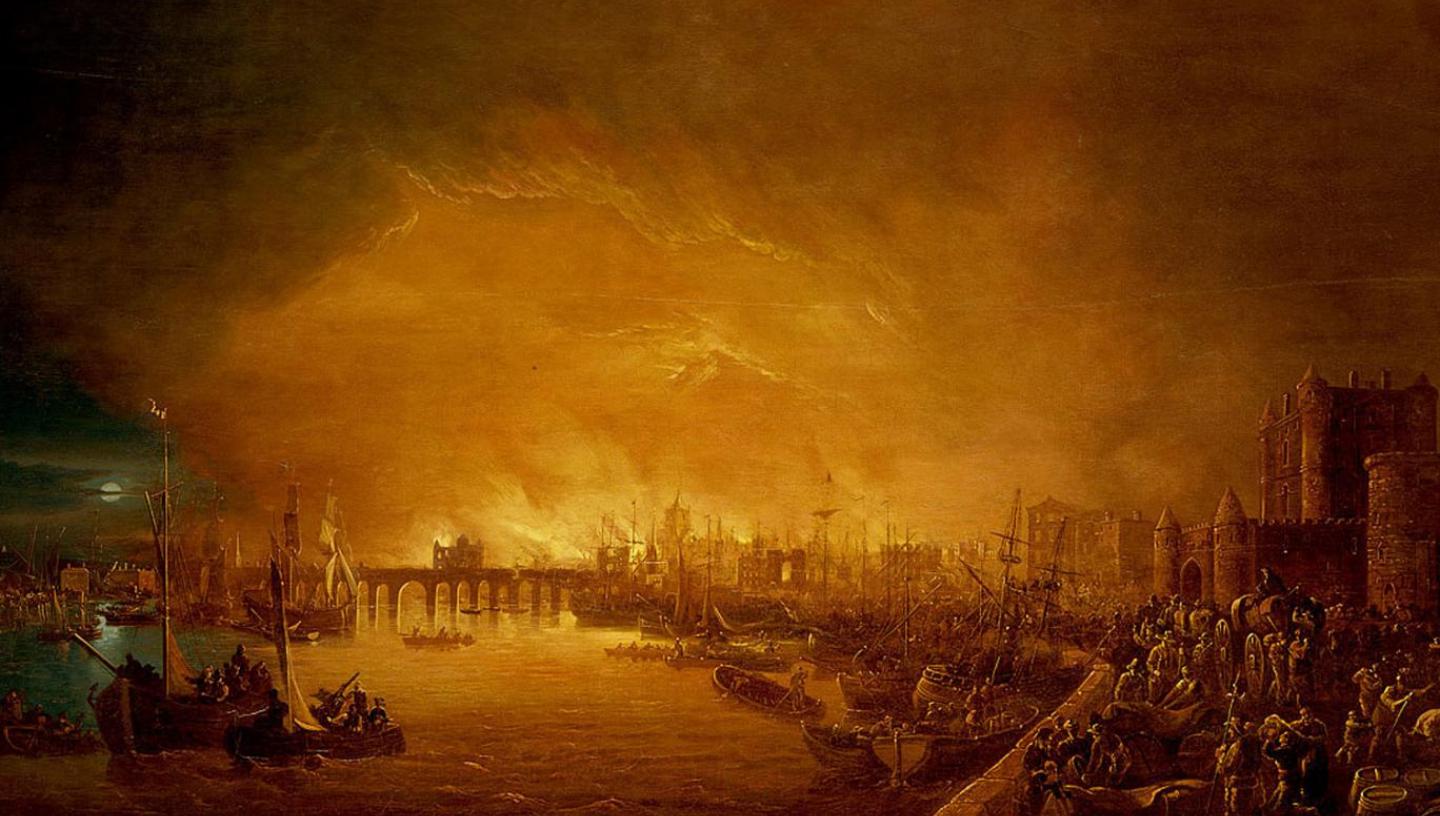The image depicts a dramatic and chaotic scene set in an older style painting, dominated by orange and yellow hues suggestive of a large fire. On the right side of the painting, we see a castle amidst the chaos, with numerous knights and soldiers, some brandishing spears, indicative of an ongoing siege. People are scattered throughout the street, many of them running, contributing to the overall sense of disorder. To the left, the painting transitions to a green-tinted section featuring water, where boats are heading towards the docks. A long pier is visible, extending toward the sea, with people standing along its border, looking out at the unfolding events. A bridge with a building on it can be seen in the distance, still mostly intact despite the surrounding turmoil. The sky is illuminated primarily by a fiery glow, though a white moon peeks through the clouds on the far left, casting a subtle light on a small section of the painting. The combination of the bright sky, the pier, and the boats, alongside the evident chaos and the castle under siege, captures a historical moment of conflict and urgency.